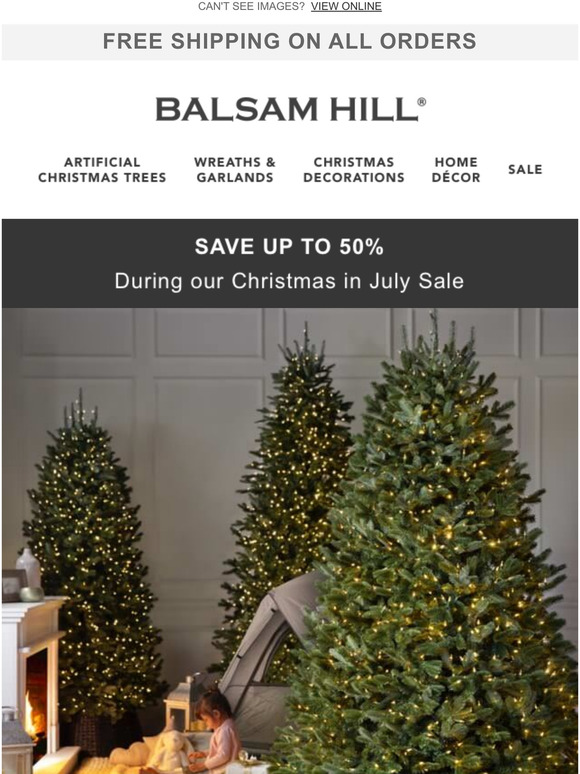The image is a screenshot from a web page largely dominated by a photograph showcasing three lush artificial Christmas trees adorned with twinkling white lights. These trees serve as the focal point, nestled in a room that features additional festive decorations dispersed across the floor and atop a nearby table. The surrounding wall is white, segmented into an arrangement of square and rectangular panels, contributing to the room's structured aesthetic.

At the very top of the web page, text in a subtle font suggests, "Can't see images? View online," followed by a light gray bar announcing, "Free shipping on all orders." Below, bold black text on a pristine white background promotes the brand and product offerings: "Balsam Hill: Artificial Christmas Trees, Wreaths and Garlands, Christmas Decorations, Home Decor, and Sale."

The primary visual centerpiece is the expansive image of the three Christmas trees, with a dark gray banner overlaying its upper portion. This banner, in prominent white text, highlights a promotional message: "Save up to 50% during our Christmas in July sale."